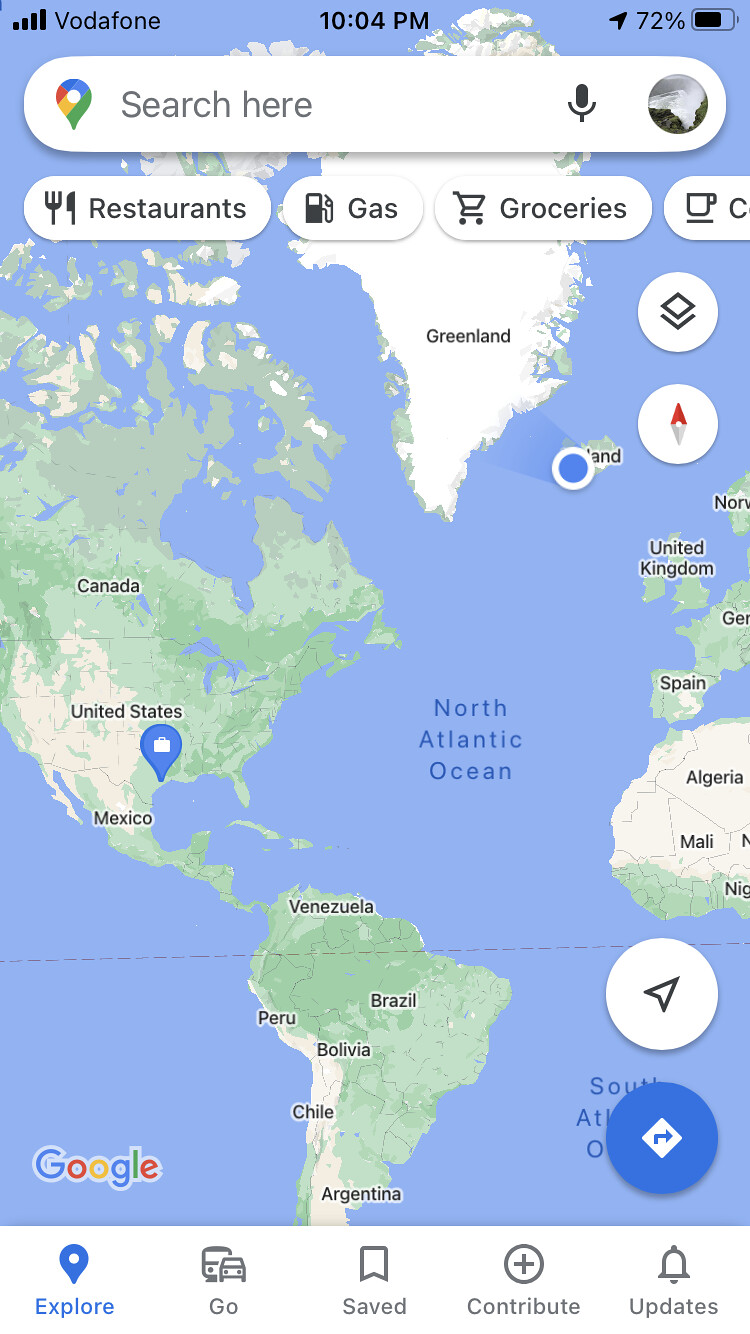In this image, the top section features the interface of a Google Maps screen, showcasing a small segment of the toolbar. Leading off is the status bar containing "Vodafone" in black text, the time displayed as "10:04 p.m." in black, and a battery icon that is 72% filled, all in black. Directly beneath this, a familiar Google search bar appears. It has the distinctive Google pin, adorned in yellow, red, blue, and green hues, alongside the prompt "Search here" in gray letters. The background of the search bar is white, and it includes a small black microphone icon for voice search options and a round icon displaying the user's profile picture.

Below the search bar, several quick-access buttons are showcased: keys for "Restaurant," "Gas," and "Groceries," each presumably leading to relevant searches. The larger portion of the image displays a geographical map with Greenland being prominently featured. This landmass is depicted with shades of green, light yellow, and white, the latter suggesting snow cover. The map extends to show the continent profiles of Canada, the United States, Mexico, most of South America, part of Africa, and the western edge of Europe which includes the United Kingdom and Spain. At the bottom of the image, "Google" is clearly labeled, cementing the platform being used.